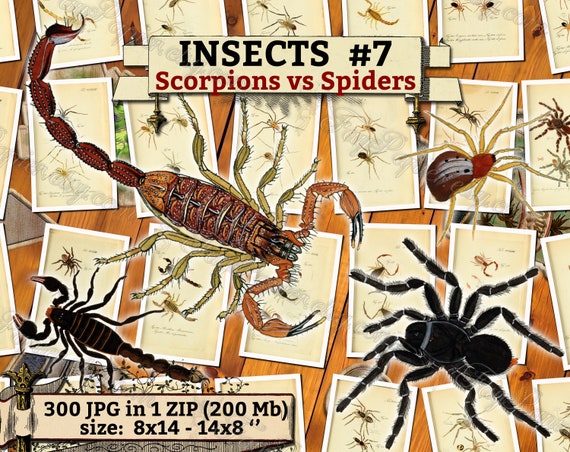This digital advertisement, designed with a cartoony illustration style, features a dramatic showdown between scorpions and spiders under the title "Insects No. 7: Scorpions vs. Spiders." The poster boasts a bold black heading with a red subheading, set against a wooden background adorned with vintage-style polaroid images of various scorpions and spiders.

Dominating the scene are a large brown scorpion and a black tarantula-like spider, depicted in confrontation at the center. Flanking these are a smaller red spider with yellow legs positioned above the tarantula, and a black scorpion aligned parallel below the larger scorpion. The layout artfully arranges these figures on a diagonal axis, adding dynamic tension to the composition.

In the bottom corner, crucial product information is displayed: "300 JPG in one zip, 200 MB, size 8 x 14, 14 x 8." This clearly indicates the availability of a digital collection featuring 300 high-quality images of scorpions and spiders, highlighting both the artistic and commercial appeal of the advertisement.